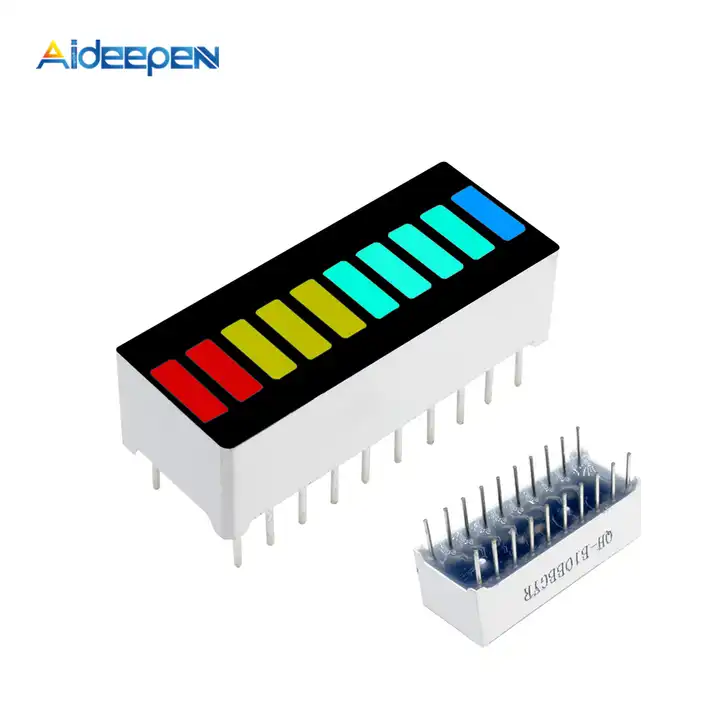This image features two distinct devices against a white backdrop. In the top left corner, a company logo displays the text "AIDEEPEN" in lowercase blue letters, where the 'A' consists of an orange triangle forming the top half and blue legs forming the bottom half of the letter. 

At the center, the main device is a white rectangular prism standing on approximately 10 to 20 thin cylindrical legs. Its top face is black and features a series of colorful rectangles in a sequence: two red, three yellow, four light blue, and the last one dark blue. Next to it, a similar device is depicted upside down, revealing its legs sticking upward and showing a translucent blue color on its upturned surface. Engraved on this inverted device is some text, although partially obscured, it includes characters like "QH-BIOBBGYR".

This detailed arrangement emphasizes the juxtaposition of the two devices and the clear branding in the upper corner, making the image both technical and visually intriguing.